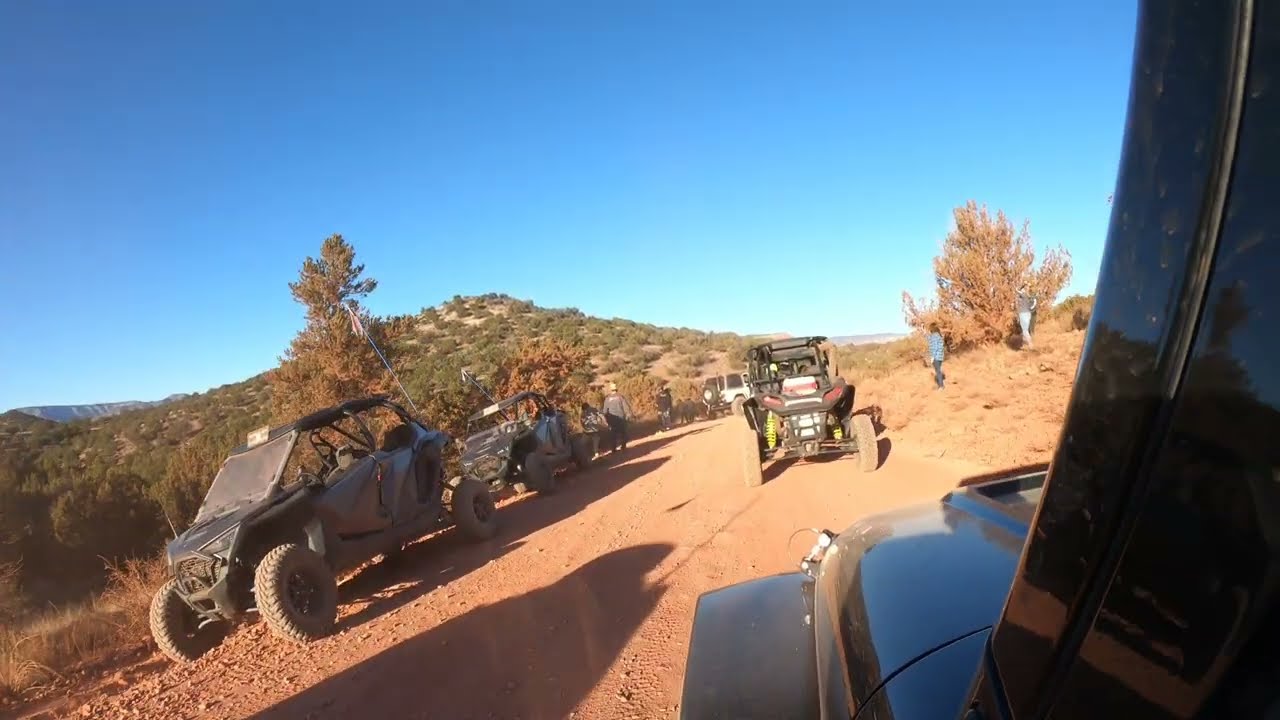The photograph captures an arid desert landscape during sunset, with a bright blue, cloudless sky above. The scene is dominated by a dirt trail lined with multiple 4x4 dirt vehicles, including several large, four-seater ATVs with big tires, and a Jeep Wrangler visible in the distance. The vehicles are parked along both sides of the path, and people are seen walking near them, with about three individuals on the left side near a grassy hill and two more on the right side, close to the vehicles. The environment features sparse, sickly trees and desert shrubs, and the terrain is marked by an orange hue typical of regions like Arizona or New Mexico. The image is taken from within one of the vehicles, providing a detailed view of the rugged and outdoor adventure setting. Shadows cast by the sun indicate it is positioned behind the photographer, contributing to the warm, sunset ambiance.